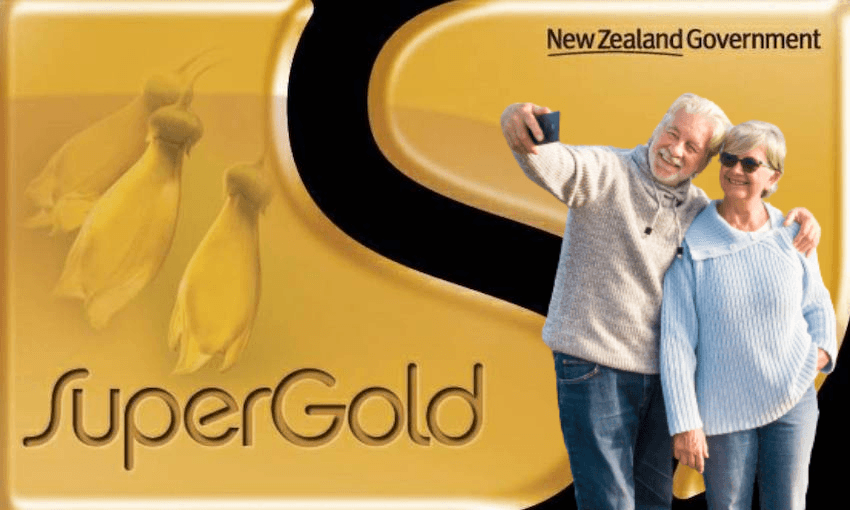In the image, a gold-toned background with subtle texture serves as the backdrop. In the top right corner, the text "New Zealand Government" is prominently displayed in a dark brown font. Below this text, towards the middle right of the image, an older couple, likely in their 60s or 70s, is taking a cheerful selfie. The man, dressed in blue jeans and a grey sweatshirt, holds a cell phone in his right hand. Next to him, the woman, wearing glasses, a light blue sweatshirt, and jeans, smiles at the camera. Through the middle of the image runs a distinctive black, swooshy, S-curved shape, giving the composition a dynamic feel. On the left side, beneath three bell-like flowers depicted in various shades of gold and not yet in full bloom, the words "Super Gold" are artistically inscribed, echoing the golden theme of the overall design.